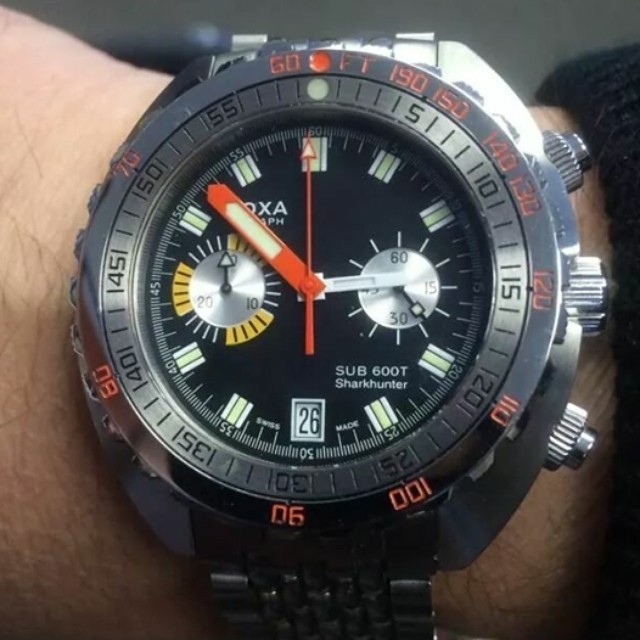This close-up image features a wristwatch with a sleek, chrome-colored casing attached to an individual's wrist. The watch face is a distinguished black, providing a striking contrast to the chrome accents. Within the main face, two smaller sub-dials are present, adding to the watch's intricate design. Instead of traditional numerical markers, the watch features minimalist square indices to denote the hours. The minute hand stands out with a chrome base highlighted by a vibrant orange detail, while the second hand is predominantly orange, finishing with a white tip. This combination of colors and design elements gives the watch a modern and sophisticated aesthetic.